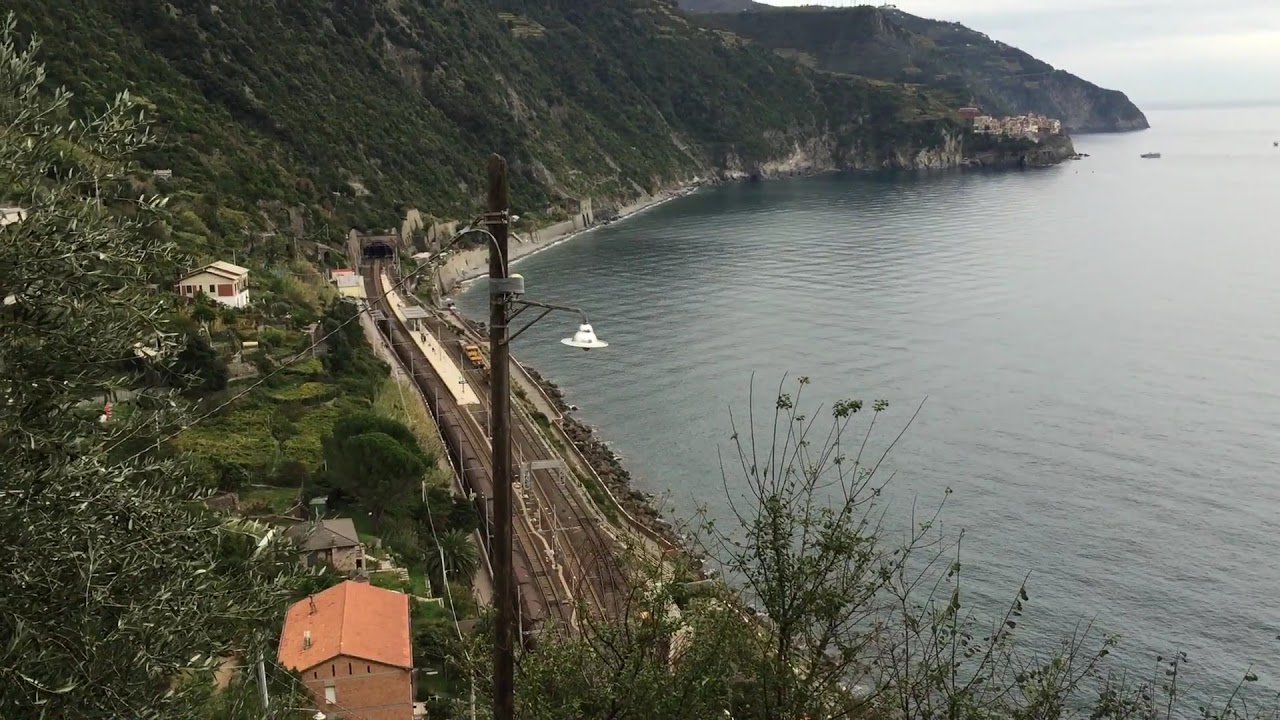This image is a color photograph taken from a high vantage point, possibly a drone, capturing a detailed and expansive view of a coastal area. To the left, the landscape is dominated by a hilly terrain thick with brush, bushes, and trees. As the hill slopes downward into a valley, three houses come into view: a prominent two-story red-bricked house, a white house, and what appears to be a gray house. Among these structures is an intricate arrangement of wide roads and train tracks; the tracks weave close to the center of the image, ultimately leading into a tunnel that burrows through the hillside.

The right side of the image reveals a tall pole with what seems to be a light fixture at the top, while an electrical or phone pole runs alongside the houses from the foreground up to the middle of the frame. Beyond the residential area, the picture transitions to a coastal setting defined by a rocky segment that arcs gracefully into a mountainous background. The bay—an almost oval-shaped body of water—spreads out, its dark gray-blue hue reflecting the sky above. Boats are visible on the water's surface, adding to the maritime feel of the scene.

Encapsulating the essence of this landscape in a realistic, representational photographic style, the image captures the serene yet complex interplay between natural and man-made elements in this picturesque coastal region.